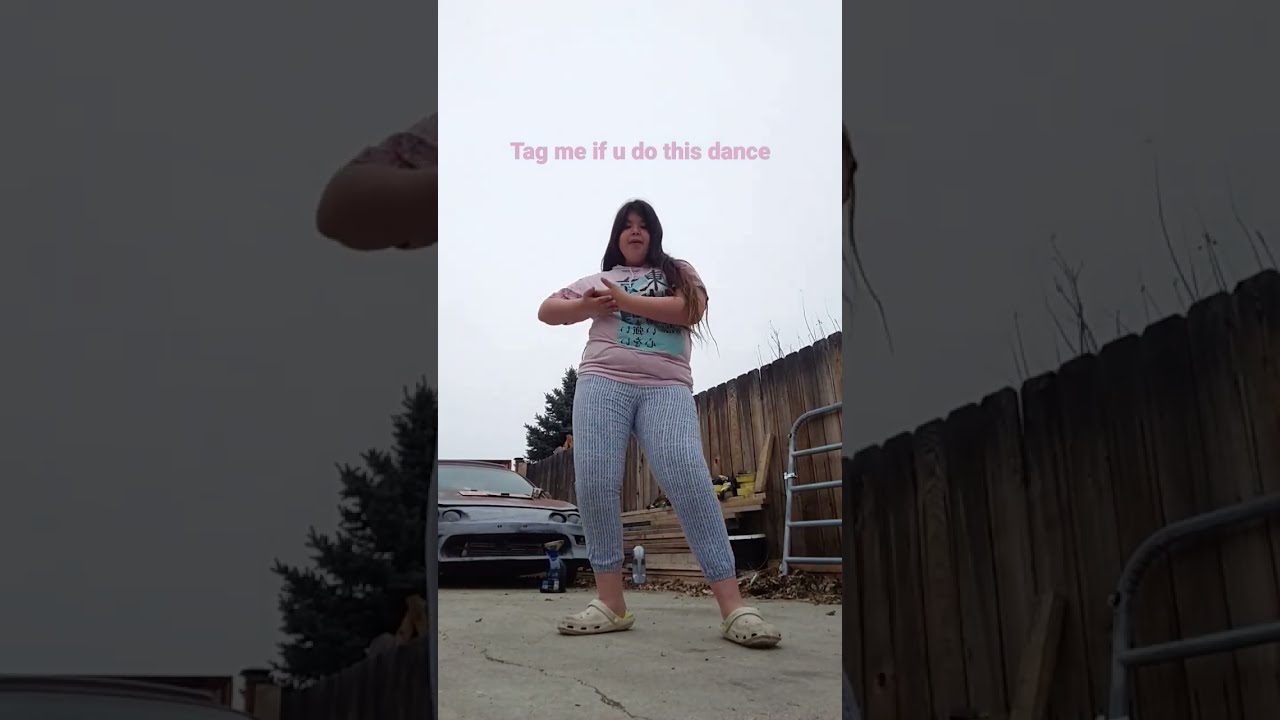In this horizontal rectangular image, the main subject is a slightly heavyset young girl centered in a narrower vertical rectangle against a predominantly cloudy grayish-white sky. She has long brown hair, and is wearing black-and-white striped leggings, a pink short-sleeved t-shirt with green and teal decoration, and white Crocs. Her hands are clasped in front of her chest as though she is performing a dance move. Above her head, the text "tag me if you do this dance" is written in light purple letters. Surrounding the central section, the left and right thirds of the image feature dimmer, zoomed-in versions of the girl's figure, emphasizing the composition. She stands on a sidewalk in front of an older car and a white-brown picket fence, suggesting an outdoor setting possibly like a backyard. The overall scene evokes a casual, playful atmosphere with its mix of everyday elements and the invitation to join in the dance.